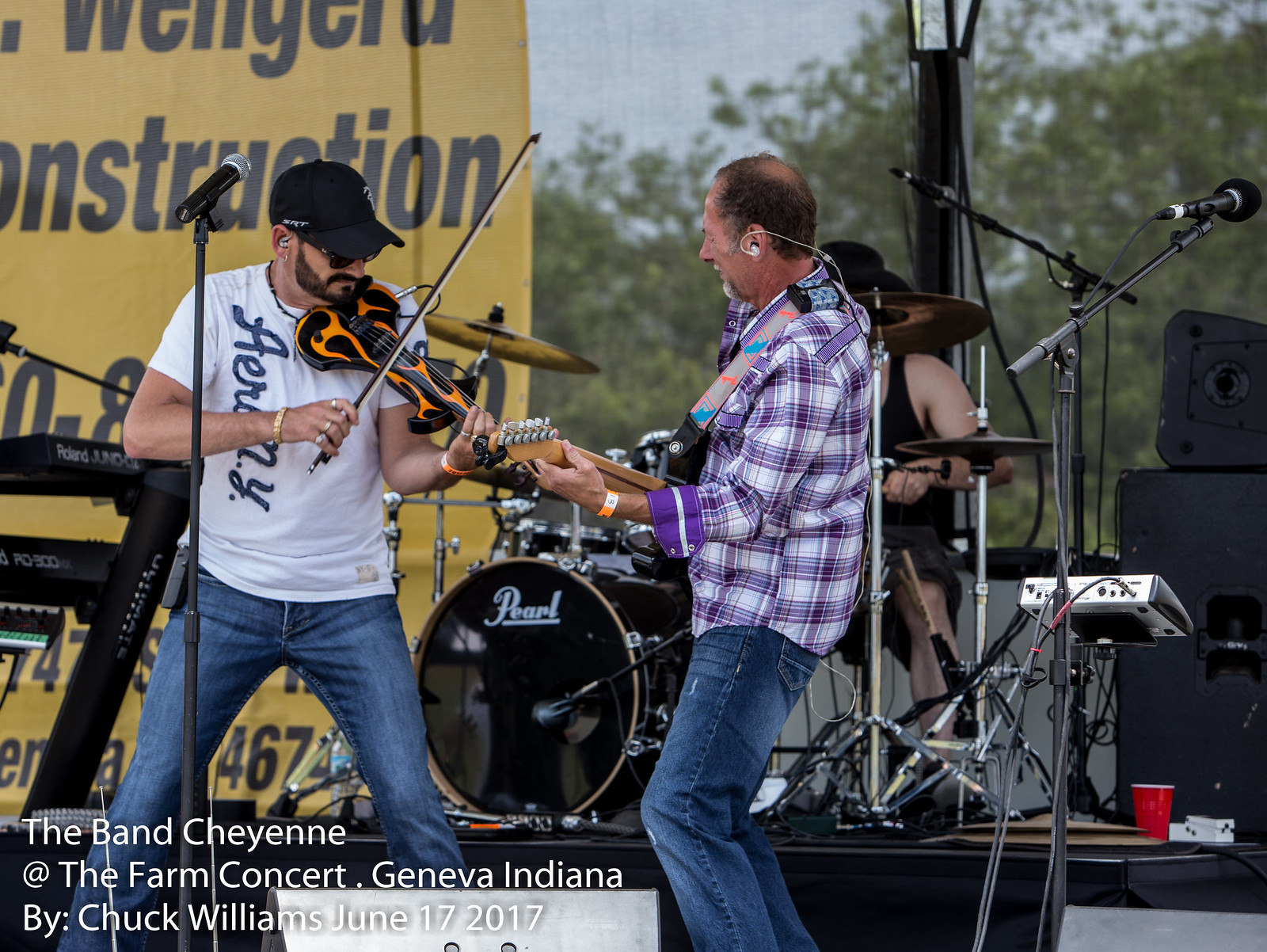In the center of the image, a vibrant outdoor concert is captured featuring three band members of Cheyenne performing at the Farm Concert in Geneva, Indiana on June 17, 2017. Two musicians are prominently positioned in the foreground. On the left, a man in a white t-shirt with vertical letters, blue jeans, a black baseball cap, and sunglasses, passionately plays an electric violin adorned with black and orange flame designs. Beside him to the right, another musician, wearing a blue and white checkered shirt and jeans, skillfully handles a guitar. Behind them, a drummer dressed in shorts, a black tank top, and a wide-brim hat, energetically plays a black drum set with the white “Pearl” logo visible on the drum face. The stage is dotted with various microphones and speakers. The bottom left corner of the image features text in white letters: "The band Cheyenne at the Farm Concert, Geneva, Indiana. By Chuck Williams, June 17, 2017." The event takes place under bright daylight, evidenced by the clear, warm lighting and vibrant colors, including shades of yellow, black, white, orange, and red, adding to the lively atmosphere of the concert.